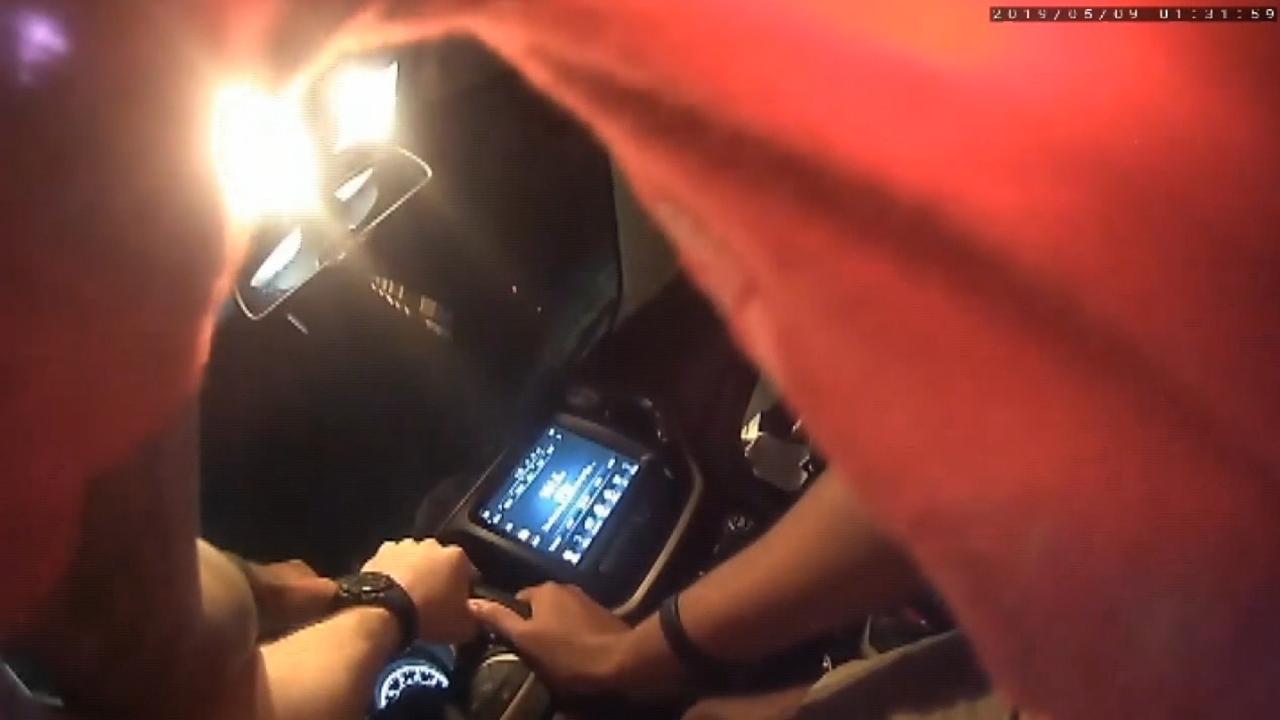The image depicts two individuals sitting in the front seat of a car, each with a hand on the steering wheel. One person wears a watch on their left wrist, while the other has a watch on their right wrist. The car interior features a brown color scheme with a black dashboard. A speedometer and a display screen are visible on the dashboard, showing radio information and music details. Above the dashboard, the windshield reveals a view of trees outside. The interior light is turned on, illuminating the seating area, and a rearview mirror is also visible. The person in the passenger seat is wearing a red shirt. In the top right corner of the image, a timestamp reads "2019/05/09," though the exact time is unclear.